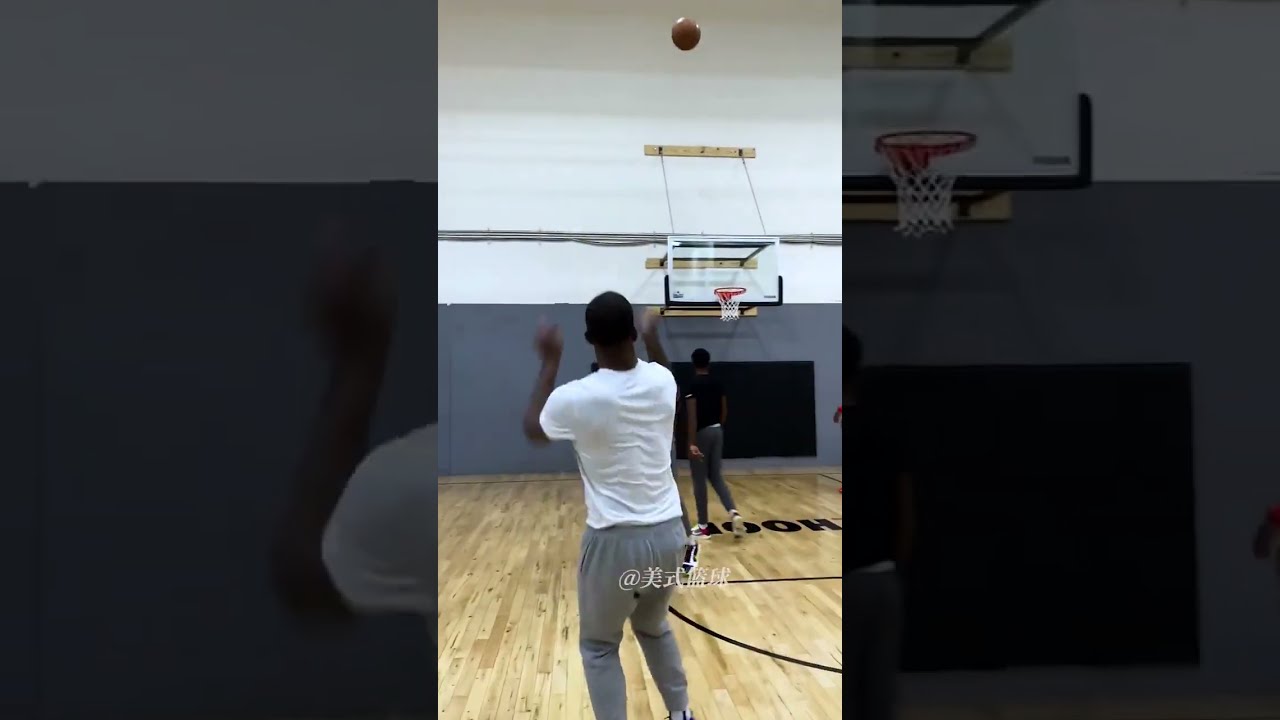In this photograph, taken on a phone, two black men are on an indoor basketball court, both facing away from the camera. The man in the foreground, wearing a white t-shirt and gray sweatpants, is captured mid-shot, with the basketball in mid-air at the top of the image. He stands just outside the center circle of the wood gym floor. Closer to the goal, another man with slightly longer hair is seen, dressed in a black t-shirt and dark gray pants. The clear backboard of the basketball hoop and the net are positioned against a wall that is gray on the bottom and white on top. The wall features visible pipes or cords running along the edges. There is unreadable text on the court and some Asian characters in the foreground. The contrast between the light wood floor and the darker surrounding edges of the photo emphasizes the action on the court.